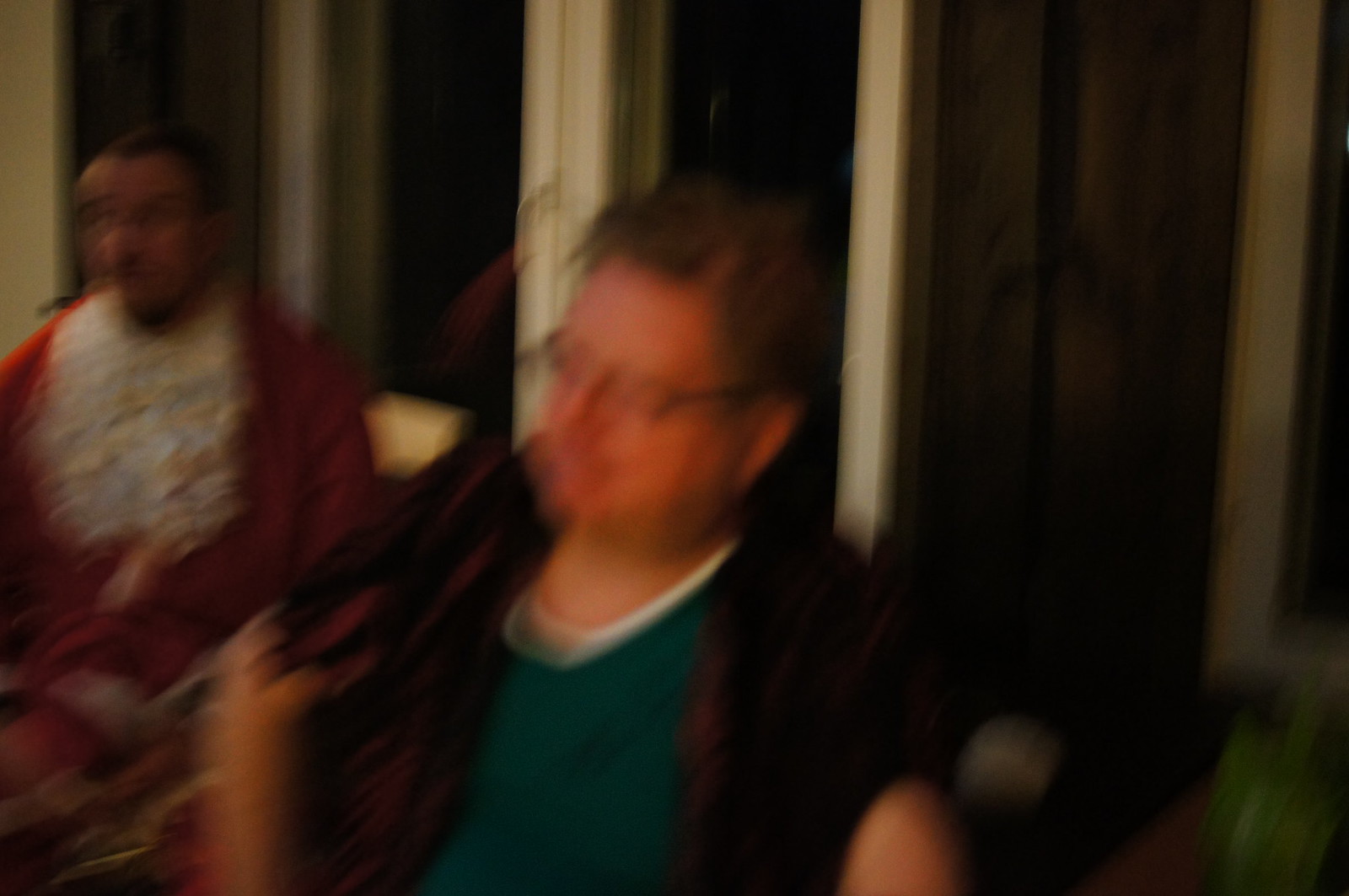A blurry and distorted photograph captures two individuals in what appears to be an indoor setting. At the center of the image is a man with short brown hair, wearing black glasses, a black shirt, and a possible white undershirt. Behind him, indistinct black blinds cover either windows or doorways. To his left stands another male, who appears to have a darker skin tone. He is dressed in a white shirt with a red jacket. Due to the blurriness, it is difficult to discern additional details about their surroundings or expressions.